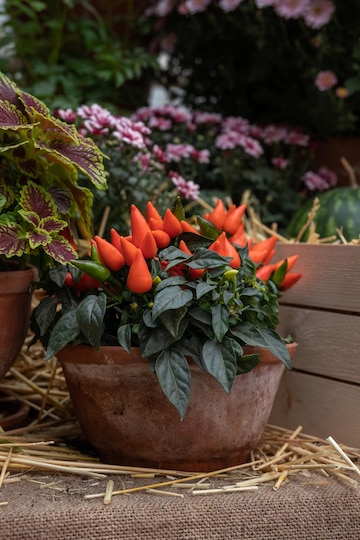This image provides a detailed close-up of a garden scene, prominently featuring a potted plant with dark green, spade-shaped leaves and numerous conical, orange objects which are likely baby carrots. This pot is made of clay, with a hint of dust over its brown surface, and it sits atop a bench covered in a mesh fabric or burlap, sprinkled with hay. Adjacent to this pot, on the left, there's another pot housing a plant with green leaves marked by purplish centers. On the right side of the scene, a glimpse of a watermelon can be seen, bordered by wooden planks running horizontally. The background showcases a vibrant display of pink flowers and green bushes, contributing to the garden's lush and lively atmosphere.